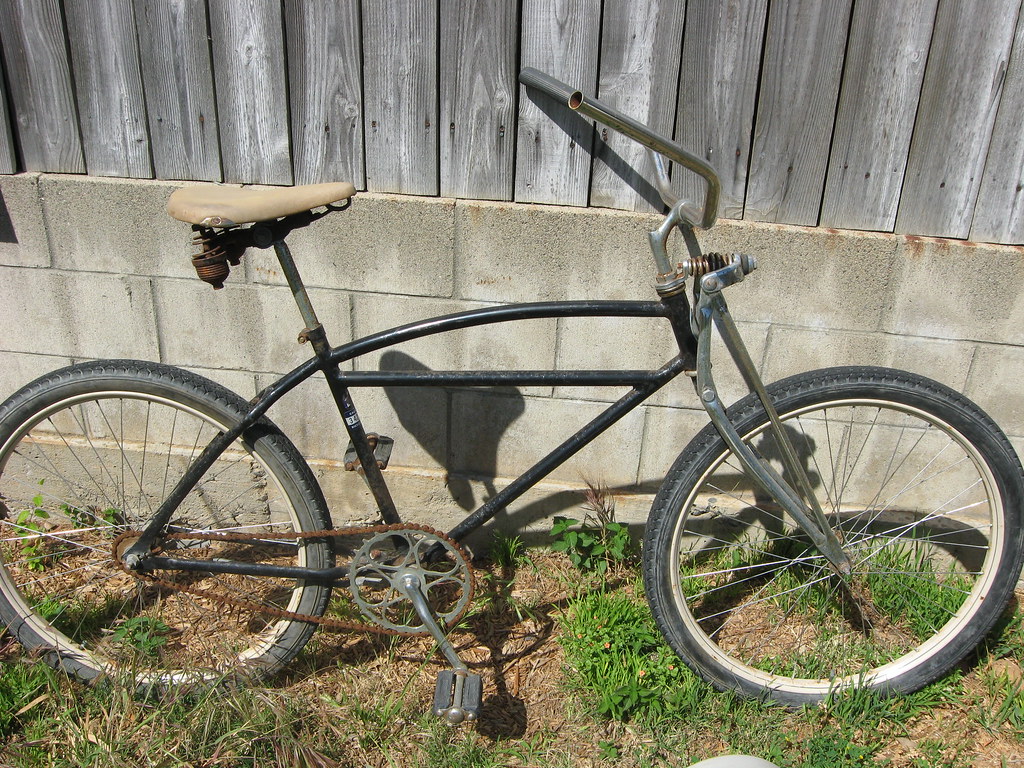This high-quality photograph captures a vintage SWIN bicycle, likely from the early 1970s, positioned outdoors against a backdrop of a weathered wooden fence with vertical slats atop a cinder block base. The bicycle, which has a black painted frame and chrome front forks equipped with a small spring, features flat tires, a rusty chain, and a worn, deteriorated cream-colored seat supported by rusty springs. The silver, dull chrome handlebars curve upward and are missing their rubber grips. The scene is set in an unkempt yard with patches of dead grass and scattered bark, highlighting the rustic and aged charm of this antique bike.